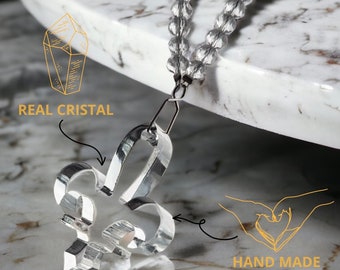The image features a detailed advertisement for a handmade crystal pendant. The pendant, crafted from a clear crystal material, is shaped like a fleur-de-lis symbol, similar to the crest used by the Boy Scouts and the New Orleans Saints logo, with a tall, rounded top and two stems that fan outwards and point downward, ending in a single point at the bottom. This crystally thick pendant is attached to a thick, round silver chain with a metal clip. The pendant and chain rest on a white marble surface that features brown lines. Above, there is a white marble shelf of the same material. Notably, the upper left-hand side of the image includes the text "Real Crystal," along with a small yellow crystal illustration. The bottom right-hand side is marked with the word "Handmade" and a drawing of two hands forming a heart. Black arrows point to these informative elements on either side of the image.